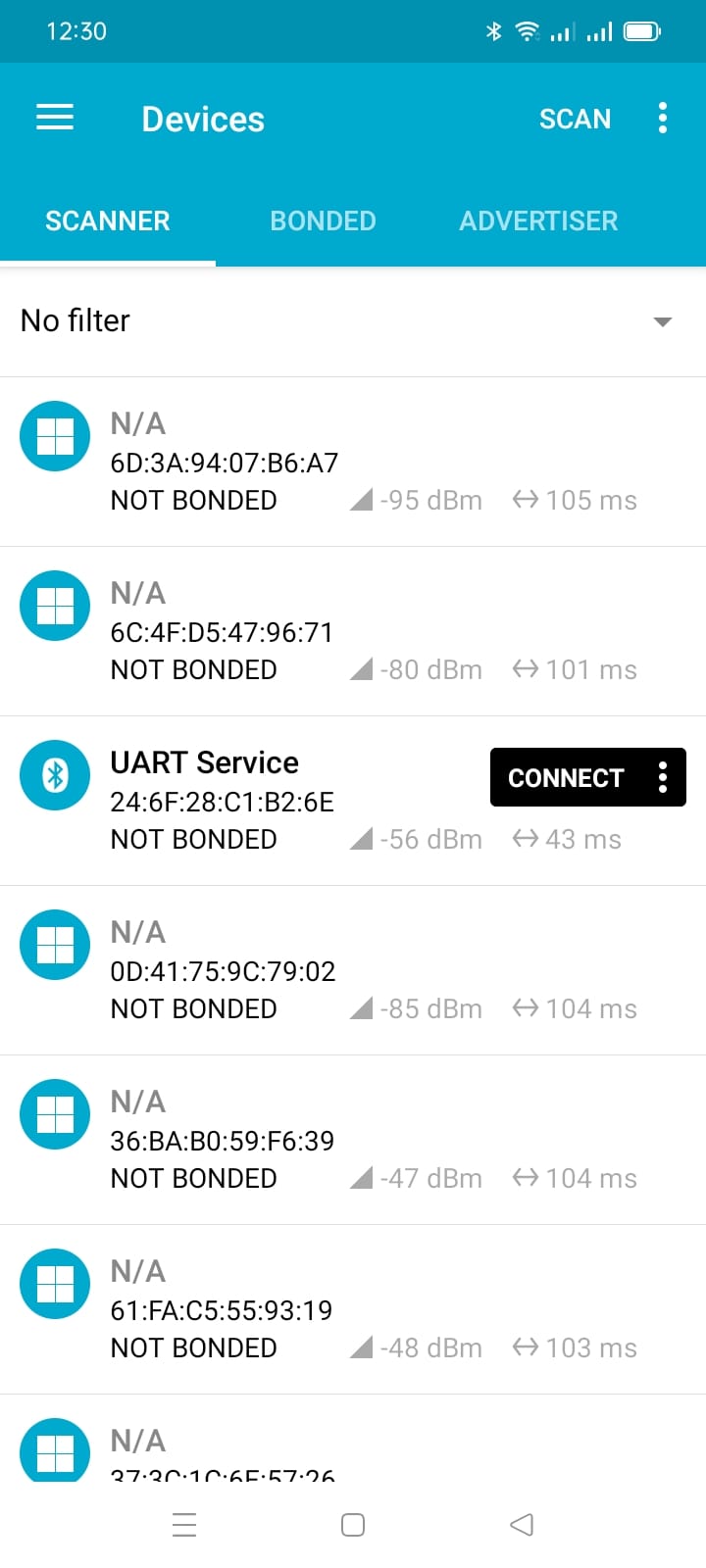This image is a detailed screenshot of an Android smartphone running a wireless device scanner application. At the top of the screen, the status bar is displayed with a dark blue background. In the top left corner, the time reads 12:30. The top right corner features icons for wireless signal strength, phone signal strength, and battery level, with the battery indicator showing approximately 70-80% charge.

Just below the status bar, a light blue box contains white text labeling "Devices" on the left and a "Scan" button with three vertical white dots on the right, indicating a menu for scanning wireless devices. Below this, there are three menu options: "Scanner" in white text (indicating it is the active option with a white underline), and "Bonded" and "Advertiser" in light gray text.

Vertically aligned below the menu options are seven entries representing different hardware devices detected on the current wireless network. Each entry features the device's name (mostly "N/A" except for one labeled "UART service"), a string of characters and numbers representing the device's MAC address, and statistics such as signal strength and distance from the scanning device.

At the bottom of the screen, a horizontal white bar displays standard Android navigation buttons, providing essential controls for the smartphone.